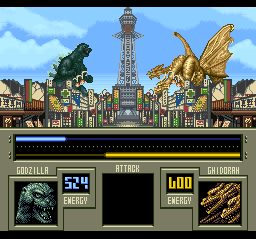The image is a digital game screenshot featuring a pixelated battle scene from a Godzilla game. Centered in a bustling town with colorful low-rise buildings, a silver structure reminiscent of a hybrid between the Eiffel Tower and the Space Needle stands tall. To the left, Godzilla, depicted in blue-green tones, is poised atop the buildings, ready for combat. On the right, a formidable golden dragon named Ghidorah, with multiple heads, faces Godzilla from a similar perch. The background showcases a serene blue sky with clouds. At the bottom of the screen, two icons representing Godzilla and Ghidorah are displayed alongside their energy levels—Godzilla at 524 and Ghidorah at 600, clearly depicting the characters' current strength in the game.